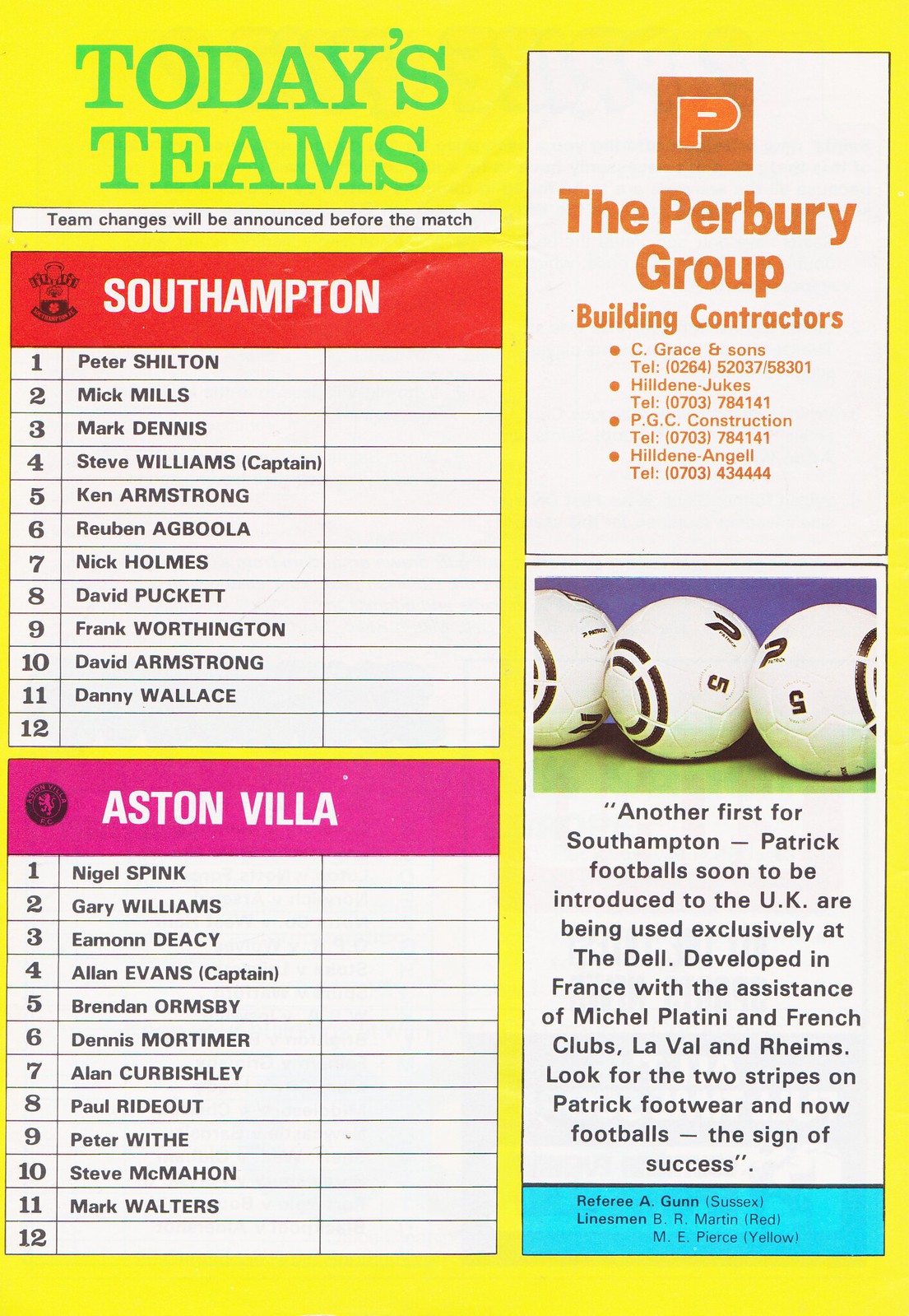The image displays a vintage magazine or pamphlet page, likely from the 70s or 80s, vigorously detailing the squads for an English football match between Southampton and Aston Villa. The page is set against a yellow background with green text announcing "Today's Teams" in the top left. Below that, in smaller black text, it notes that "Team Changes will be announced before the match."

The team listings are prominently featured with Southampton's lineup under a red headline and white text. The squad includes: 1. Peter Shilton, 2. Mick Mills, 3. Mark Dennis, 4. Steve Williams (Captain), 5. Ken Armstrong, 6. Reuben Agboola, 7. Nick Holmes, 8. David Puckett, 9. Frank Worthington, 10. David Armstrong, and 11. Danny Wallace.

Adjacent, Aston Villa's lineup is presented on a pink background with white text: 1. Nigel Spink, 2. Gary Williams, 3. Iman Deasy, 4. Alan Evans (Captain), 5. Brendan Ormsby, 6. Dennis Mortimer, 7. Alan Curbishley, 8. Paul Rideout, 9. Peter Wythe, 10. Steve McMahon, and 11. Mark Walters.

In the top right corner is an advertisement for the Perbury Group of Building Contractors, identifiable by an orange rectangle featuring a white-bordered 'P' along with contact details. The bottom right corner contains a white rectangle featuring three photographed soccer balls on a green floor with a blue background, alongside a promotional quote: "Another first for Southampton, soon to be introduced to the U.K. or being used exclusively at the Dell. Developed in France with the assistance of Michel Platini and French clubs Laval and Reims. Look for the two stripes on Patrick Footwear, and now footballs, the sign of success."

At the bottom, a small blue rectangle details the match officials in black text: "Referee: A. Gunn (Sussex), Linesmen: B.R. Martin (Red) and M.E. Pierce (Yellow)."